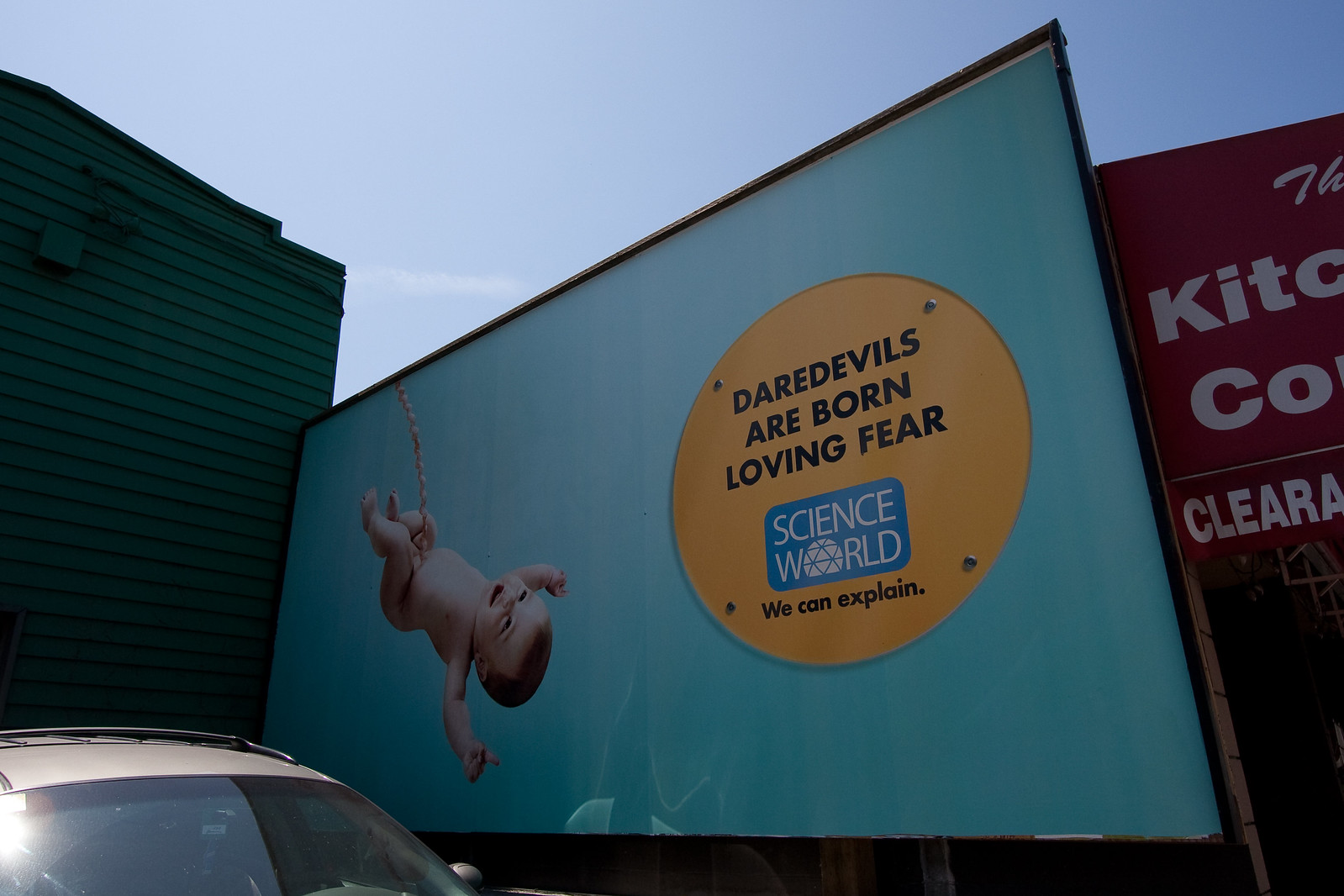The image captures a vibrant outdoor scene featuring a colorful advertisement sign. The main sign, set against a bright blue background, reads, "Daredevils are born loving fear." The striking visual centerpiece is a cheerful baby hanging upside down by a rope, with its arms raised and mouth open in apparent delight. Positioned against a green building, the sign stands out prominently. Adjacent to it, there is a red sign that partially reads "Kitchen" and "Clearance," with a "Thank you" message at the top. A parked car is visible next to the sign. The sun is shining, indicating a clear, bright day, suggesting that the image is likely an advertisement for a business in the area.